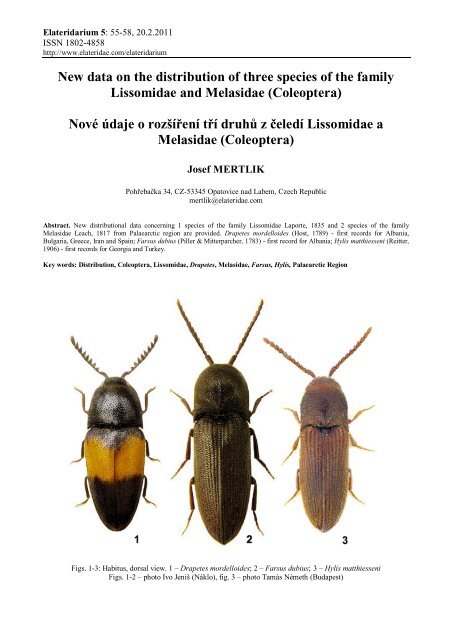The image is an information sheet featuring detailed descriptions and images of three beetle species from the families Lysomidae and Melissidae of the Coleoptera order. At the very top, in small text, it reads "alerterdarium 55-58.220.0.2011," followed by "ISN SSN 1802-4858" and an unreadable website address. Below this, in large black letters, it states "New data on the distribution of three species of the family Lysomidae and Melissidae Coleoptera," with a translation in another language beneath it. The author's name, Joseph Mertlick, is prominently displayed, followed by an abstract in small print: "New distributional data concerning one species of the family Lysomidae Laporte, 1835, and two species of the family Melasidae Leach, 1817, from the Paleo-Arctic region are provided." 

The graphic showcases three hard-shelled beetles, labeled 1, 2, and 3, with descriptions beneath each. Beetle 1 is dark brown with a yellow stripe across its back and has six legs and antennae. Beetle 2 is the largest, dark brown with a textured shell, also with six legs and longer antennae. Beetle 3 is a lighter tan with shades of gray, similar in structure to Beetle 2 but smaller, with six legs and matching antennae.